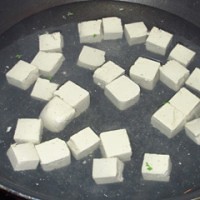The image depicts a black pot filled with water, showcasing approximately 30 to 40 white cubes floating within it. These cubes appear to be roughly cut and slightly uneven in shape, resembling tofu. The water seems to be boiling, indicated by the heat suggested in the descriptions. A close-up shot fills the entire square frame of the photograph, leaving no visible background except for a very dark, flat gray color. One of the cubes notably has a small piece of green on it, which might be an accidental inclusion.